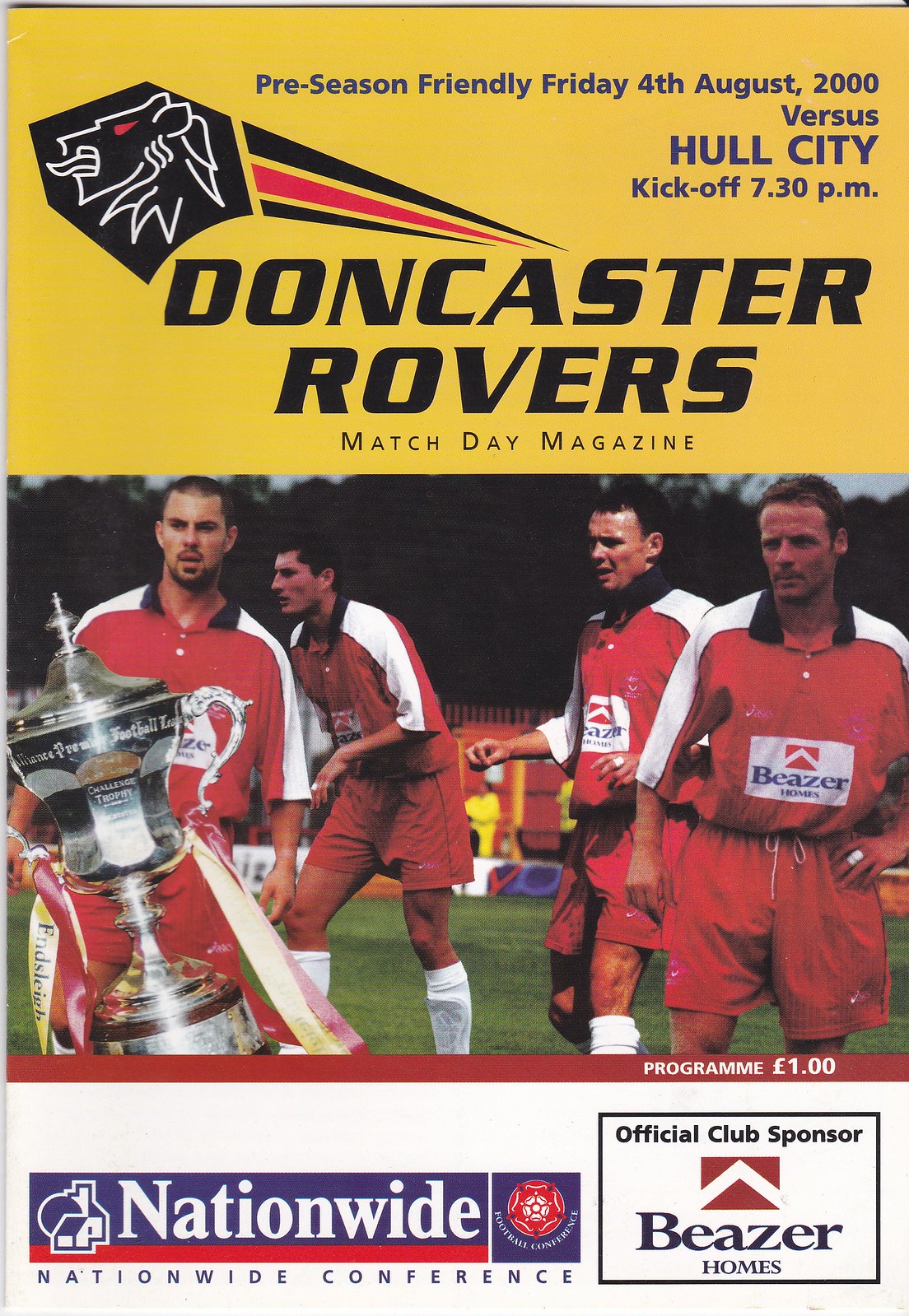This is the cover of the Doncaster Rovers Matchday Magazine for a pre-season friendly against Hull City, scheduled for Friday, 4th August 2000, kickoff at 7:30 PM. The cover features a detailed photograph of four players in red uniforms with shin guards, standing on a soccer field with trees visible in the background. A prominent silver trophy is positioned in the lower left corner of the image. The magazine's header includes black text reading "Doncaster Rovers Matchday Magazine" alongside a lion logo with its tongue out. Below the photo, two advertisements are visible alongside logos for the Nationwide Conference and official club sponsor, Beezer Homes. The magazine is priced at one pound. The scene is set outdoors on a green pitch with predominantly red, white, yellow, black, and shades of blue colors.